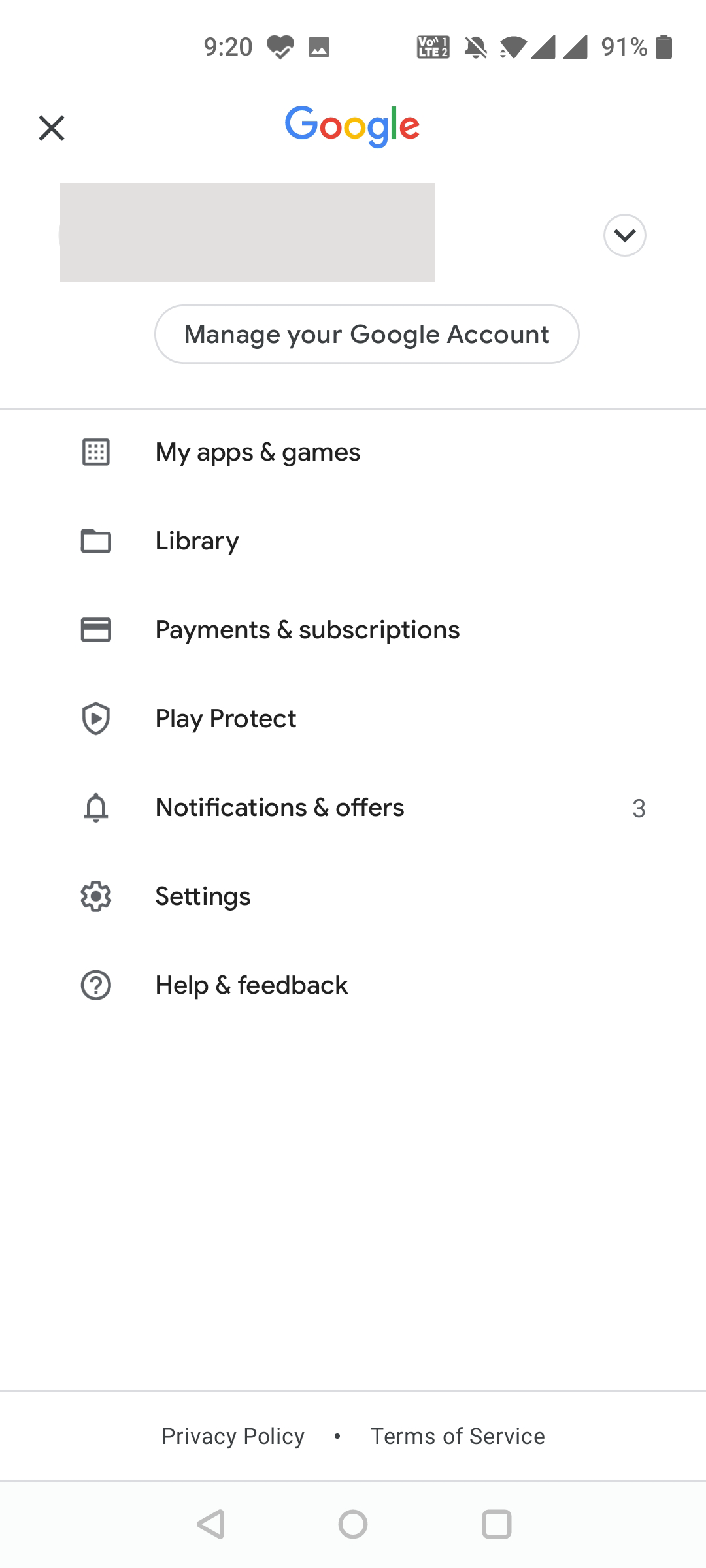This screenshot, taken from a mobile device, showcases the account settings page of a Google account. In the upper right-hand corner, details such as the battery life and the time are visible, confirming that this is indeed a mobile screenshot. Dominating the upper section of the screen is the iconic Google logo, spelled out in its signature rainbow colors. Notably, certain sensitive details, such as the account holder's name and Gmail address, have been censored for privacy.

Centered on the page is a prominent button labeled "Manage your Google Account." Directly below this button, an array of options for managing the account are displayed. These include:

- My apps & games
- Library
- Payments & subscriptions
- Play Protect
- Notifications & offers (with a notification counter showing the number three)
- Settings
- Help & feedback

These options allow the user to navigate different aspects of their Google account with ease.

Towards the bottom of the screenshot, there are two important links: "Privacy Policy" and "Terms of Service," providing users with quick access to Google's legal and user-policy documents. Additionally, an 'X' button located in the upper left-hand corner allows the user to easily exit the account settings page if needed.

Overall, this detailed depiction gives a comprehensive view of the Google account settings interface on a mobile device, highlighting its various functionalities and features.